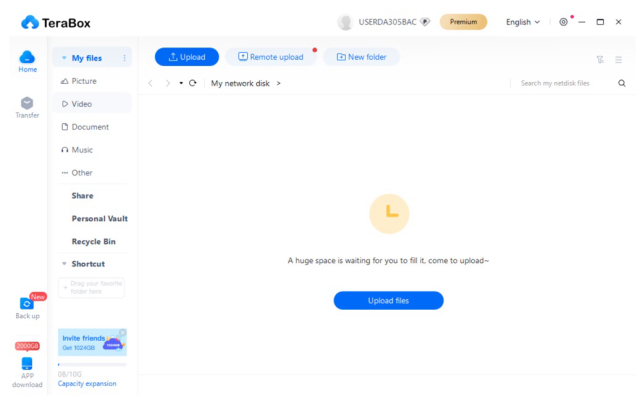The screenshot appears to be from the upload section of a website, specifically featuring Terabox. On the left-hand side at the top, the Terabox logo or label is displayed. Beneath this, there are various headings listed sequentially: "My Files," "Picture," "Video," "Document," "Music," and "Other." Additionally, in bold text, the categories "Share," "Personal Vault," "Recycle Bin," and "Shortcut" are also visible, indicating different sections within the interface.

In the center of the page, there's a prominent yellow clock icon, accompanied by a motivational message that reads, "A huge space is waiting for you to fill it. Come to upload." Directly below this message, a noticeable blue button with white text invites users to "Upload Files."

Overall, the interface is designed to guide users through organizing and uploading their files efficiently with clear categorical sections and an inviting call-to-action button.